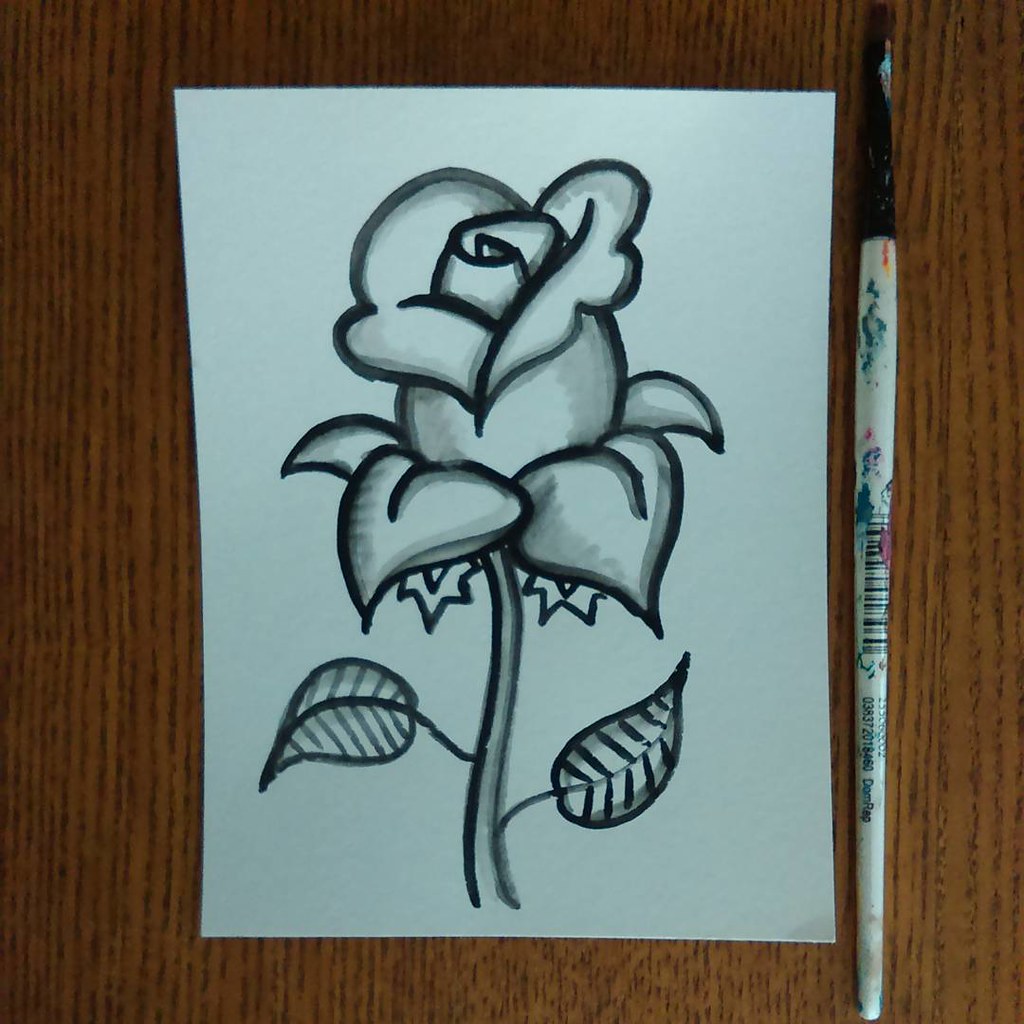The photograph captures a piece of artwork resting on a brown hardwood table with prominent vertical wood grain. The artwork is a black and white drawing of a fully bloomed rose on a sheet of white paper, occupying approximately 80% of the sheet. The rose, detailed with minor shading along its stem, leaves, and the edges of the flower, features four leaves around the bloom at the top. This delicate line drawing appears to have been created using either a large permanent marker or watercolors. To the right of the paper lies a white-handled paintbrush with multicolored paint splotches and a barcode still attached. The brush is positioned vertically, but its bristles are cut off from the image. The composition is simple and there is no additional text, signatures, or other elements present in the photograph.